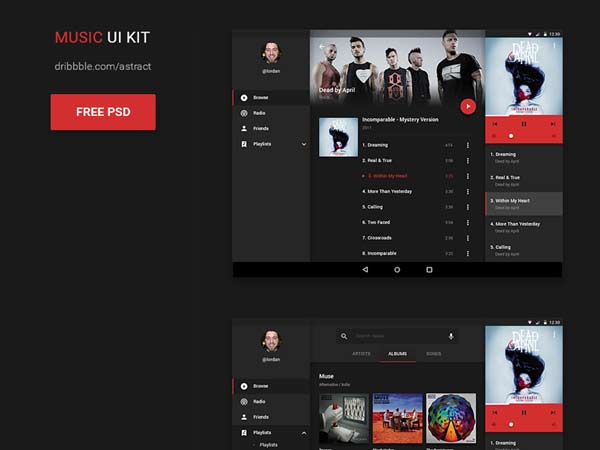Here is a detailed and cleaned-up caption for the given image description:

---

The image showcases a screen from a design labeled "Music UI Kit" available on dribbble.com by ASTRACT. The primary interface is a sleek, modern music player presented in a free PSD format. Dominating the left side is a prominent red button with white text, and adjacent to it is a high-resolution mock-up of various screens. 

Central to the display is a glamour shot of a five-member male band, each sporting graphic t-shirts with at least one member featuring a mohawk and others donning sleeveless attire. Their edgy style is further accentuated by their shaved hairstyles. 

At the top left, there is a user icon followed by an unreadable menu directly below. Beneath the band image, a music player interface takes center stage. It includes a notable red play button, an indication that at least eight songs are available, with the third track highlighted in red, suggesting it is currently playing.

To the right, there seems to be a graphic of a person with their hair flying upwards, possibly labeled as "Dead Daphne" or "Dead April," although the text is unclear. The interface accurately demonstrates the music player's features, including a detailed progress bar and playback controls such as pause, end song, and begin song options. 

The interface also highlights five different options, with the third option currently selected. Below this primary section, the screen transitions into a diverse collage of other photos mixed in, giving a dynamic feel to the interface. This additional content is categorized under the "Albums" tab, showing at least three previously released albums from the band, adding depth to the user experience.

--- 

This detailed caption provides a comprehensive overview of the various elements in the design, highlighting key aspects of the user interface and the artistic presentation of the music player.